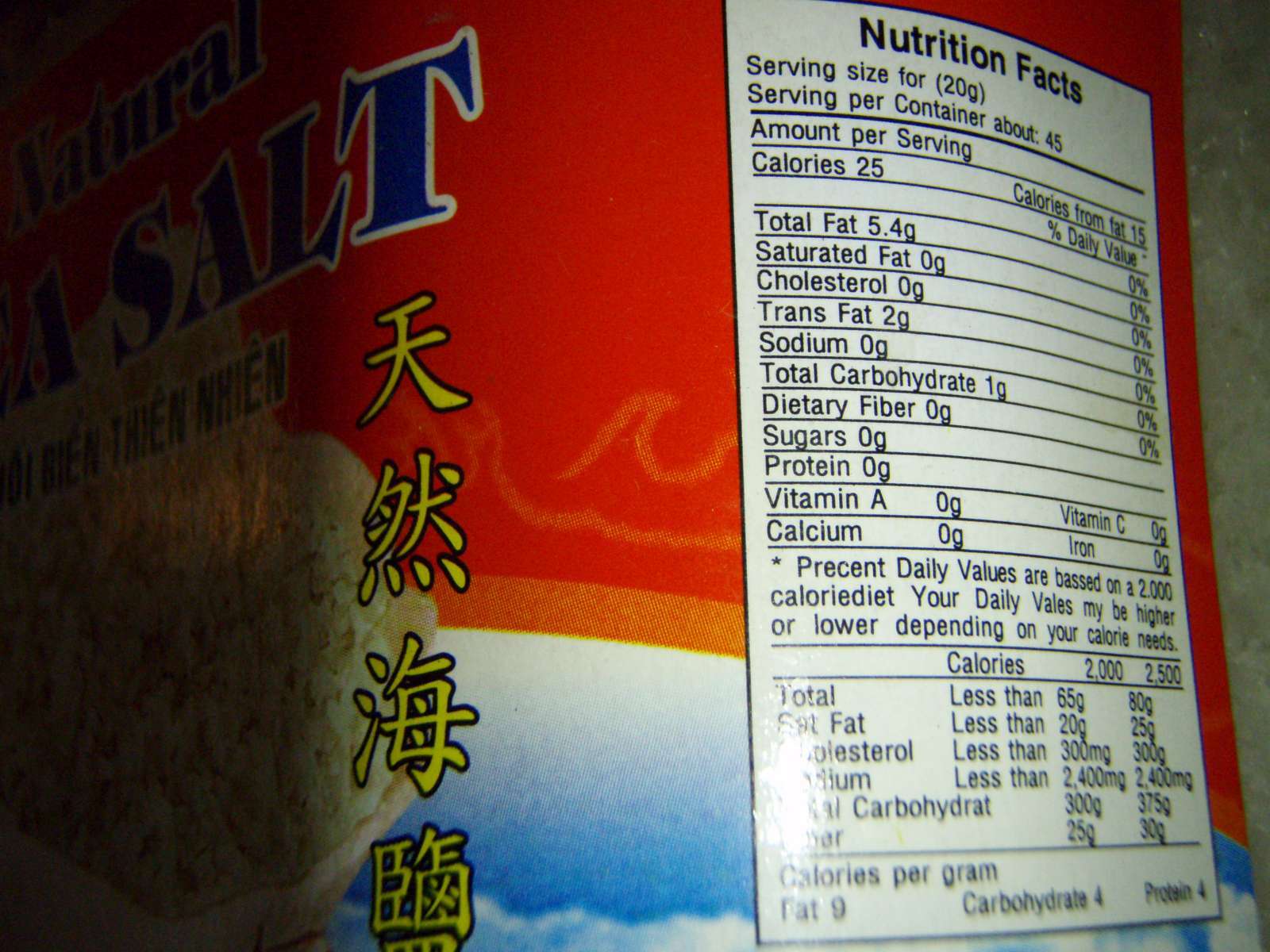This is a detailed close-up photograph of an Asian food packaging, specifically ramen noodles, captured at an angle that reveals both the front and side panels. The packaging features a vibrant combination of colors with the top portion in red, an orange line below it, and blue clouds at the bottom. The word "SALT" is prominently displayed in large, blue, capitalized letters outlined in white. Beneath this, there are Asian characters in yellow font and a partial image of the food against a white background. 

The side panel displays a large, white, vertical box with the heading "Nutrition Facts" in black, where only the 'N' and 'F' are capitalized. The nutrition information is detailed and reads as follows: serving size is 20 grams, with approximately 45 servings per container. Each serving contains 25 calories and 15 calories from fat. The daily values listed are: total fat at 5.4 grams (0%), saturated fat at 0 grams (0%), cholesterol at 0 grams (0%), trans fat at 2 grams (0%), sodium at 0 grams (0%), total carbohydrate at 1 gram (0%), dietary fiber at 0 grams, sugars at 0 grams, protein at 0 grams, and no significant amounts of vitamin A, vitamin C, calcium, or iron. These percentages are based on a 2000 calorie diet, with daily values that may vary depending on individual dietary needs. 

There is a slight glare from the lighting on the lower left part of the nutrition label, adding a reflective shine to the packaging.